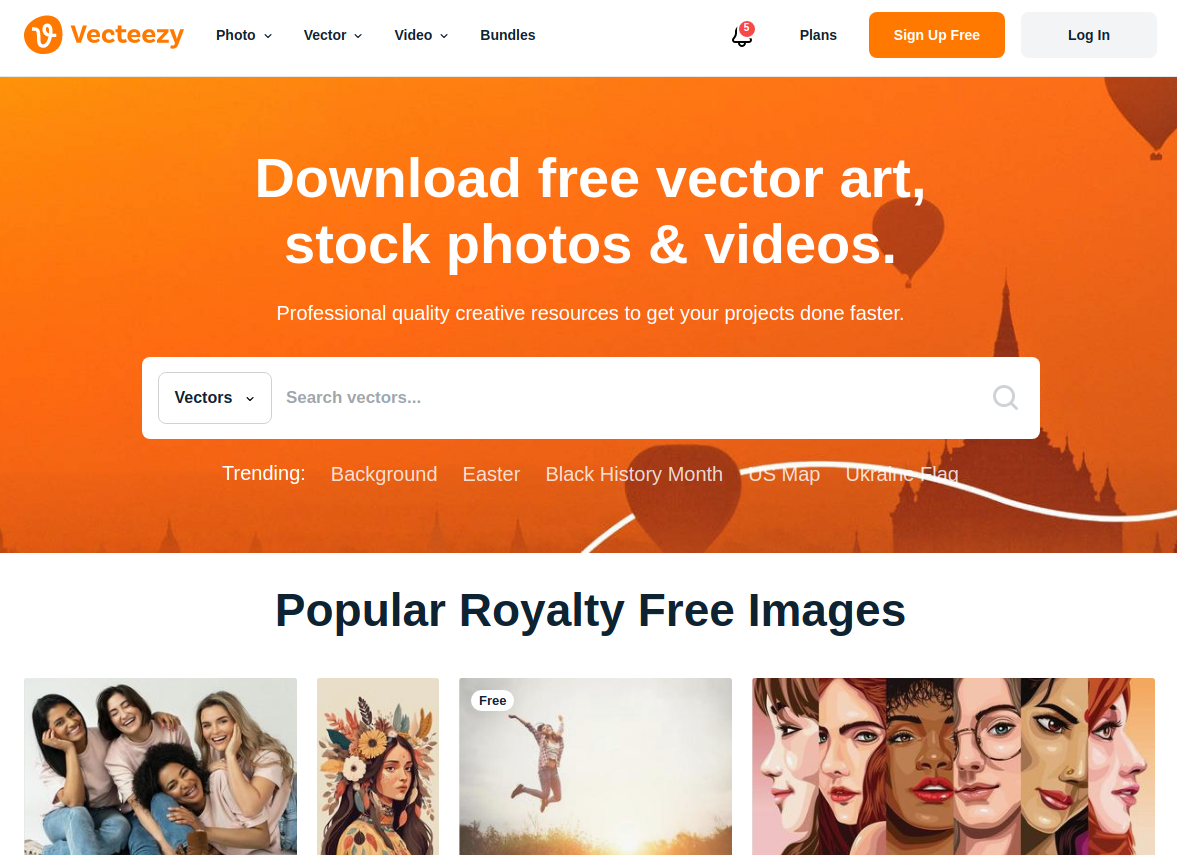The image features a clean and user-friendly interface of a website called "Vectizy". In the top left corner, the Vectizy logo is displayed with an orange circle and a white "V" next to the brand name in orange. Alongside the logo, there are four navigation tabs labeled "Photo," "Vector," "Video," and "Bundles."

On the top right side, an icon indicates 5 notifications. Next to this are links for "Plans," and additional icons for a pattern with two variations. There are also options to "Sign up free" and "Login," where "Sign up free" is highlighted in orange and "Login" is in grey.

Centered at the bottom of the image, there's a prominent tagline: "Download free vector art, stock photos, and videos. Professional quality creative resources to get your projects done faster." Below this, there is a white search bar with the placeholder text "Search vectors."

Further beneath the search bar, trending keywords are listed in white text against an orange background, including "background," "Easter," "Black History Month," "US Market," and "Ukraine Flag." The section labeled "Popular Royalty Free Images" follows, showcasing four images side by side, featuring various subjects. Portraits of people are interspersed with other artistic visuals. The entirety of this content sits on a white background, enhancing readability and user navigation.